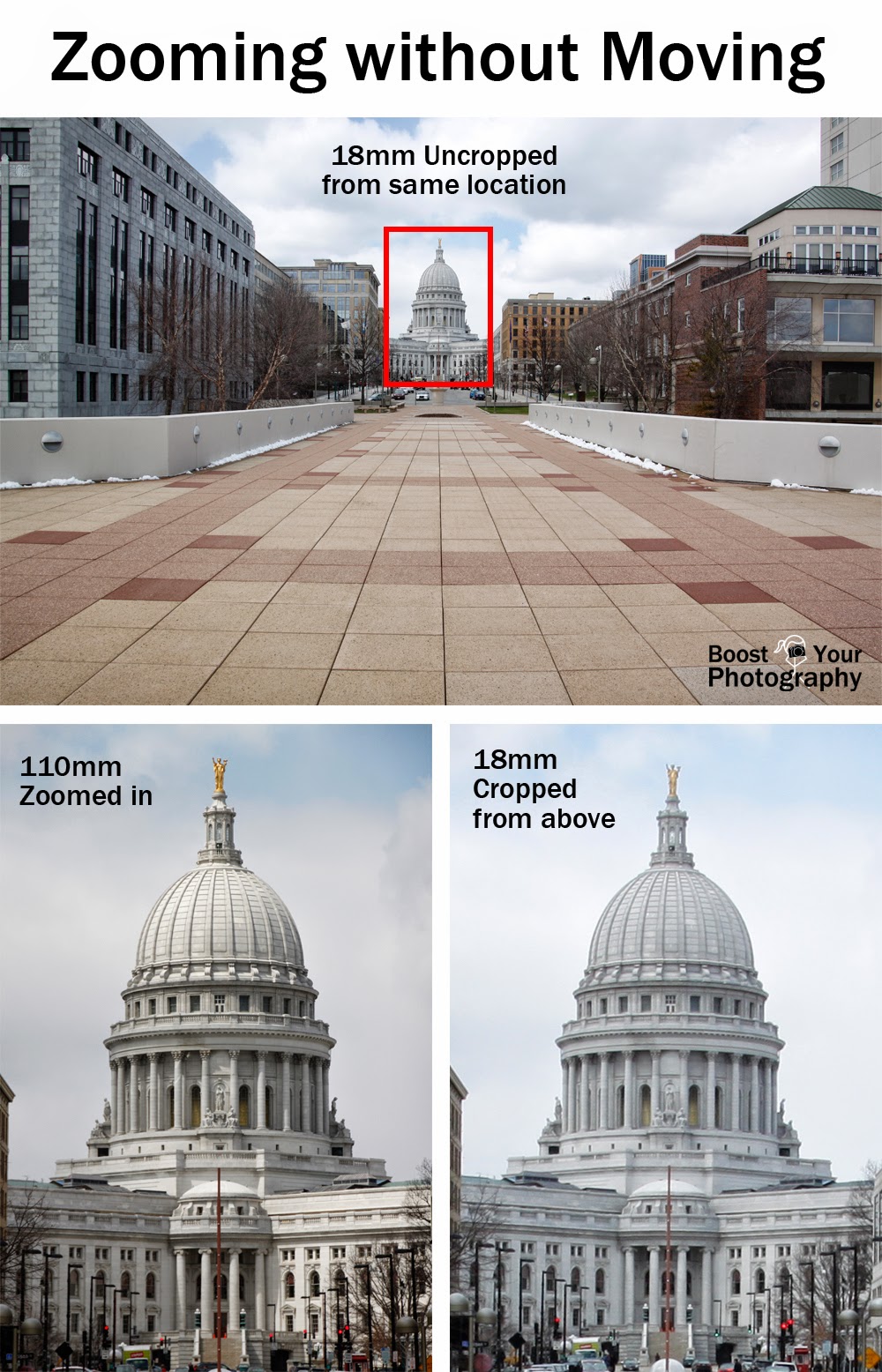The image is a composite of three color photographs with descriptive text, arranged to form an overall portrait orientation. The upper half features a landscape photograph of a cityscape capturing a red tiled pathway leading to a Capitol building with a distinctive dome. This top image has a mix of light tan and dark brown tiles, with buildings lining the edges. Text at the top of this photograph reads, "18mm uncropped from same location," and a red rectangle highlights the Capitol building's dome. In the bottom right corner, there is a black logo with the text "boost your photography," and a small white camera icon.

Below the upper photograph, the image is divided into two side-by-side photographs, both zoomed in on the Capitol building's dome but displaying different annotations. The left photograph, labeled "110mm zoomed in," shows the dome in darker tones, while the right photograph, labeled "18mm cropped from above," presents the dome in brighter, more vibrant colors, matching the top image. 

Overall, the piece combines elements of representational realism in color photography with graphic design and typography, visually illustrating the effects of zooming without moving.